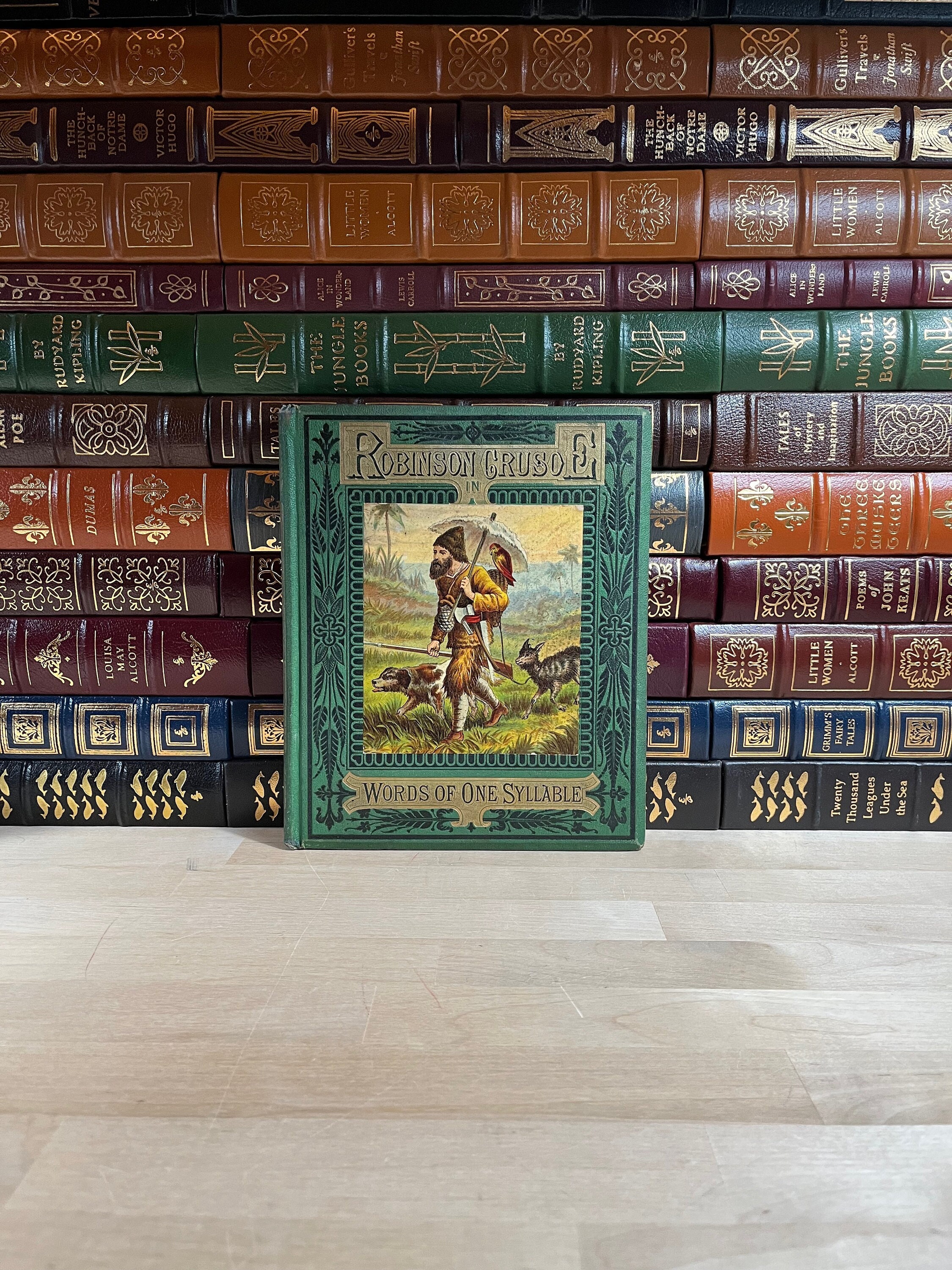The image showcases a collection of books stacked together, resting on what appears to be a light beige tiled surface. Although the exact location of the surface is unclear due to the zoomed-in nature of the image, the tiles have a super light beige shade, hinting that they might be flooring. The spines of the books are adorned with gilt lettering, and their vibrant colors range from navy blue, blue, burgundy, brown, orange, green, to a lighter brown. Notably, one book, in particular, catches the eye as it is laid horizontally across the backs of the others. This book has a green cover, decorated with darker green leaves, and features the title "Robinson Crusoe, In Words of One Syllable" prominently on its spine.